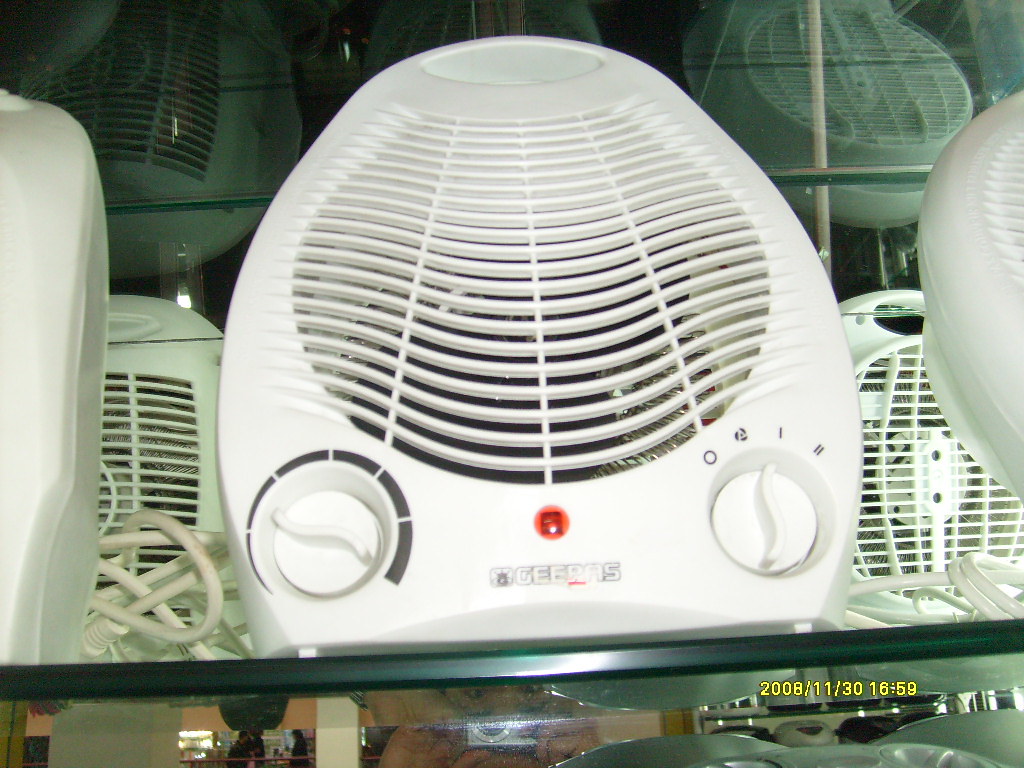This photo captures a store display featuring multiple white G-E-E-R-A-S branded desk fans, each with two white knobs at the base: the left for intensity and the right for power and settings. The fans are positioned on a glass shelf with a reflective glass back, creating a mirrored effect of the fans and revealing the presence of the individual taking the photograph, visible through the reflection of their eyes and silver digital camera. The central fan, highlighted, features a rounded top and a distinctive red light centered between the two controls. The black text "G-E-E-R-A-S" appears at the bottom of the fan, slightly faded, possibly indicating that these could be refurbished or lightly used fans. A date and time stamp in yellow text, "2008/11/30 16:59," is situated in the bottom right corner of the image. The entire setup, with its pristine arrangement and clean appearance, suggests a second-hand or wholesale store environment.